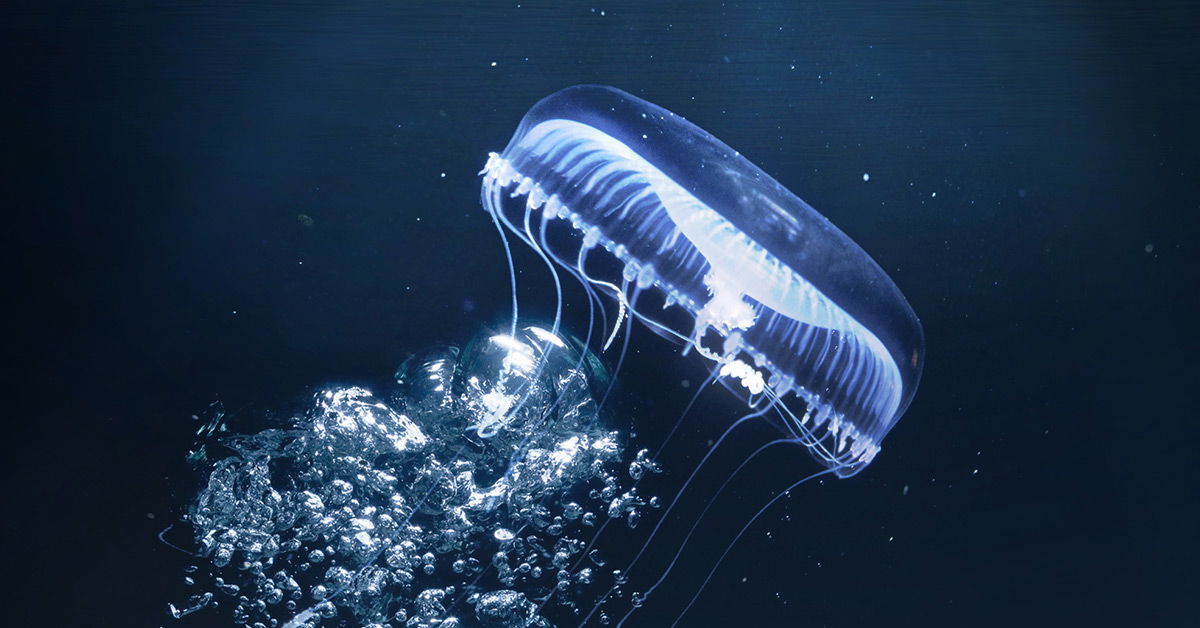In this high-definition underwater photograph, a large jellyfish is seen swimming gracefully upwards and to the right. Dominating the center of the image, the jellyfish displays a dark blue, rounded dome with a bright white underside. Its delicate, thin tentacles trail beneath, framed by a dramatic commotion of silvery bubbles of various sizes that extend from just underneath the jellyfish towards the bottom left corner of the image. The surrounding water is a deep, almost midnight blue that slightly lightens near the top of the jellyfish, giving the creature an ethereal, almost glowing appearance. Scattered around the jellyfish and even underneath it, towards the bottom right of the image, are numerous little white dots, adding to the enchanting, otherworldly scene. There are no people or other animals present, emphasizing the jellyfish's solitary majesty against the vast, dark backdrop of the ocean.